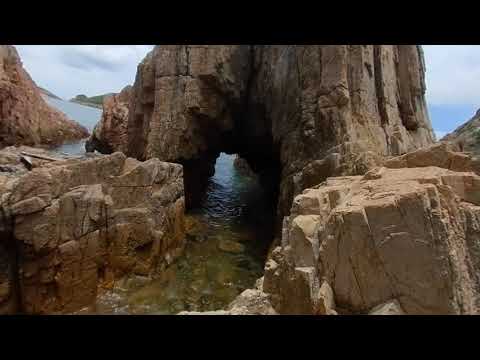The photograph captures a striking natural waterway carving through a monumental rock formation. Over time, the water has sculpted a passage, creating a tunnel-like or cavernous canal that flows through the bottom center of a large, rugged rock. The rock itself exhibits a textured, craggy surface, predominantly light brown with patches of gray. Flanking the waterway are sharply angled rocks, forming a canyon-like entryway into the more extensive, darker gray rock formation behind. This massive structure features an open arch, allowing water to flow from one end to the other, guiding the viewer's eye through to a broader body of water that stretches into the background. 

The scene is imbued with earthy tones, mostly brown and gray, with specks of green from distant mountains and a hint of blue from the sky and distant ocean or wide bay. The sky above varies from light blue to gray, with one visible white cloud adding contrast. There are no people in sight, emphasizing the natural, untouched beauty of the landscape. The overall lighting suggests it is midday, highlighting the intricate details of the rock formations and the serene flow of the water through the natural archway into the vast expanse beyond.